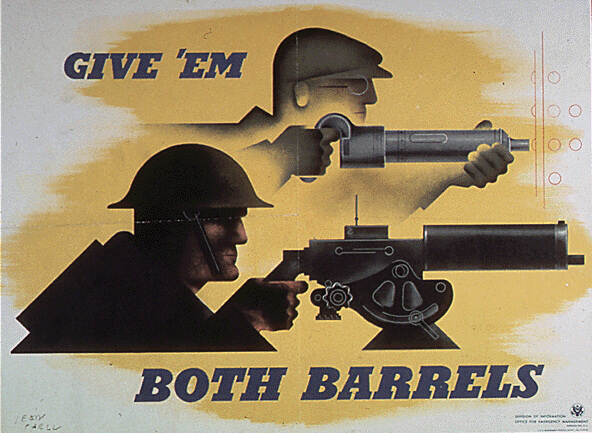This image is a rectangular, wide, textured paper poster that appears to have been folded, as evidenced by a noticeable crosshair-type fold in the center, dividing it into four sections. The overall style evokes an old military wartime poster. The poster features a man on the top sporting a beret-style newsy hat and goggles, holding a long, elongated gun with a silver barrel aimed ahead. Below him is a soldier with a round military helmet, depicted in a side profile. This soldier is Caucasian, gripping a black machine gun with a tilting mechanism that allows it to point upwards or downwards. Both men are facing and aiming their weapons to the right, and the image gives off a dimly lit, silhouette-style appearance with hints of skin visible.

Text on the poster includes a dark blue "GIVE 'EM" in the upper left corner and a prominent "BOTH BARRELS" in blocky, all-capital text at the bottom center. Background features include a gold splatter behind the two men. Additionally, the bottom right displays some logos, while the bottom left bears a signature, further anchoring the vintage and authoritative feel of this well-worn poster. The dominant colors in the image are black, gray, light yellow, off-white, and brown, harmonizing with the military theme.